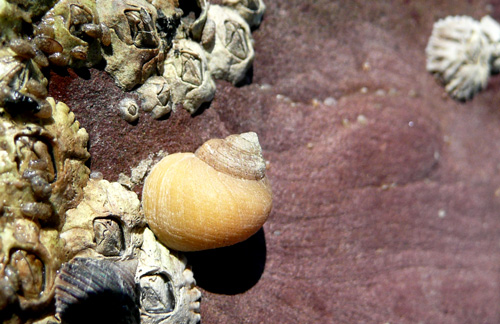This detailed image, presented in a landscape orientation, captures an array of marine elements resting on a slightly curved stone surface that fades from purple to brown. Centered slightly to the left, there lies a prominent, large conch shell with a light gold hue and a spiral top. Surrounding it, predominantly on the left side, are various seashells, coral formations, and barnacle-type sea life, creating a clustered and textured aggregation. The sandy, pebbled stone surface backdrop exhibits a dark red to purple coloration, enhancing the organic contrast. In the upper right corner, a blurred stone or shell object subtly frames the composition, adding depth and a touch of mystery. The image likely gives an underwater impression, as there appears to be a waviness, suggesting it might be photographed through water, possibly even within a fish tank setting.